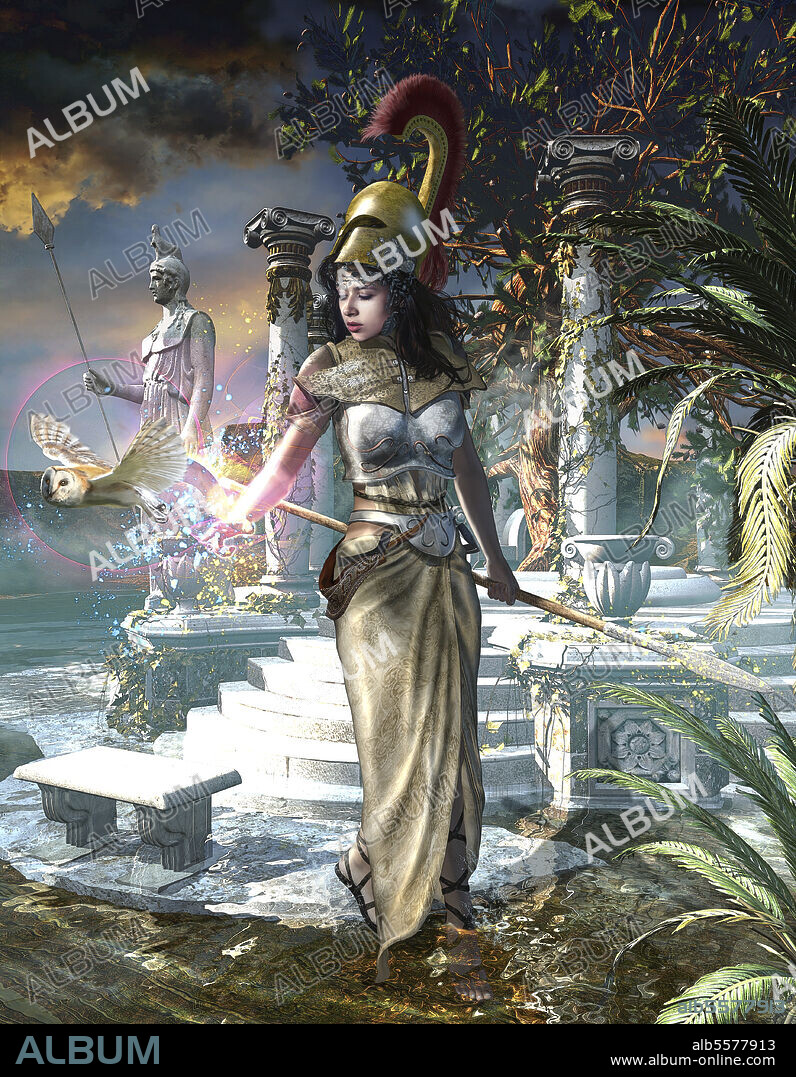The image depicts a vibrant, fantastical ancient Greek scene rendered in computer graphics. Dominating the foreground is a warrior woman, poised with determination, clad in a gleaming plate armor chest piece and a flowing, loose-fitting skirt. Atop her head rests a Spartan-style hoplite helmet. Her right hand wields a spear, whose tip glistens with glittering particles. 

In an evocative moment, she reaches out towards an owl, with multicolored sparks elegantly tracing a path from the bird to her outstretched hand, creating a mystical connection between them. Behind her, a grand staircase ascends from the ground, flanked by majestic, ivy-draped columns that lend an ancient, overgrown beauty to the scene. 

In the background, to her right, stands a regal statue of a man holding a spear, adding to the classical ambiance. The entire composition blends elements of mythology and history, brought to life with rich detail and vibrant hues.